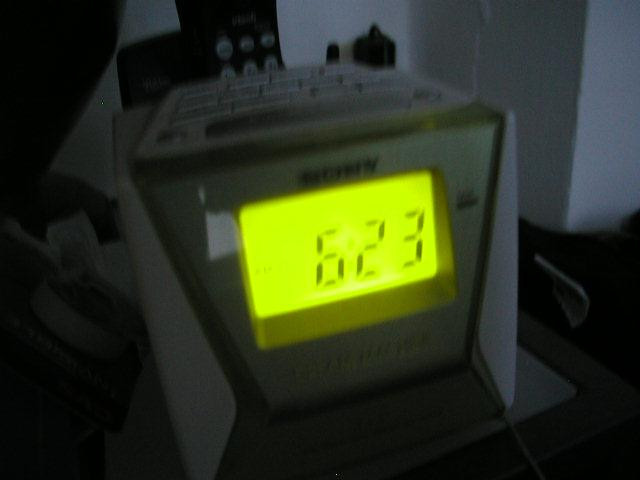This image depicts a square Sony alarm clock in a low-resolution, dark setting. The clock, which occupies the majority of the picture, has a lime-yellow-green digital display showing the time as 6:23, with 'PM' indicated on the left side. Despite the blur, the Sony brand name is discernible above the display. The top of the alarm clock is crowded with approximately 14 buttons, which appear to serve various functions such as setting the time and alarm. The alarm clock's body is mostly white with a potential black frame and is placed on a brown, likely bedside table. Behind the clock, there is a black, cordless phone reminiscent of 1990s models. The background features a white-painted, cement wall, contributing to the overall grainy and dark atmosphere of the image.